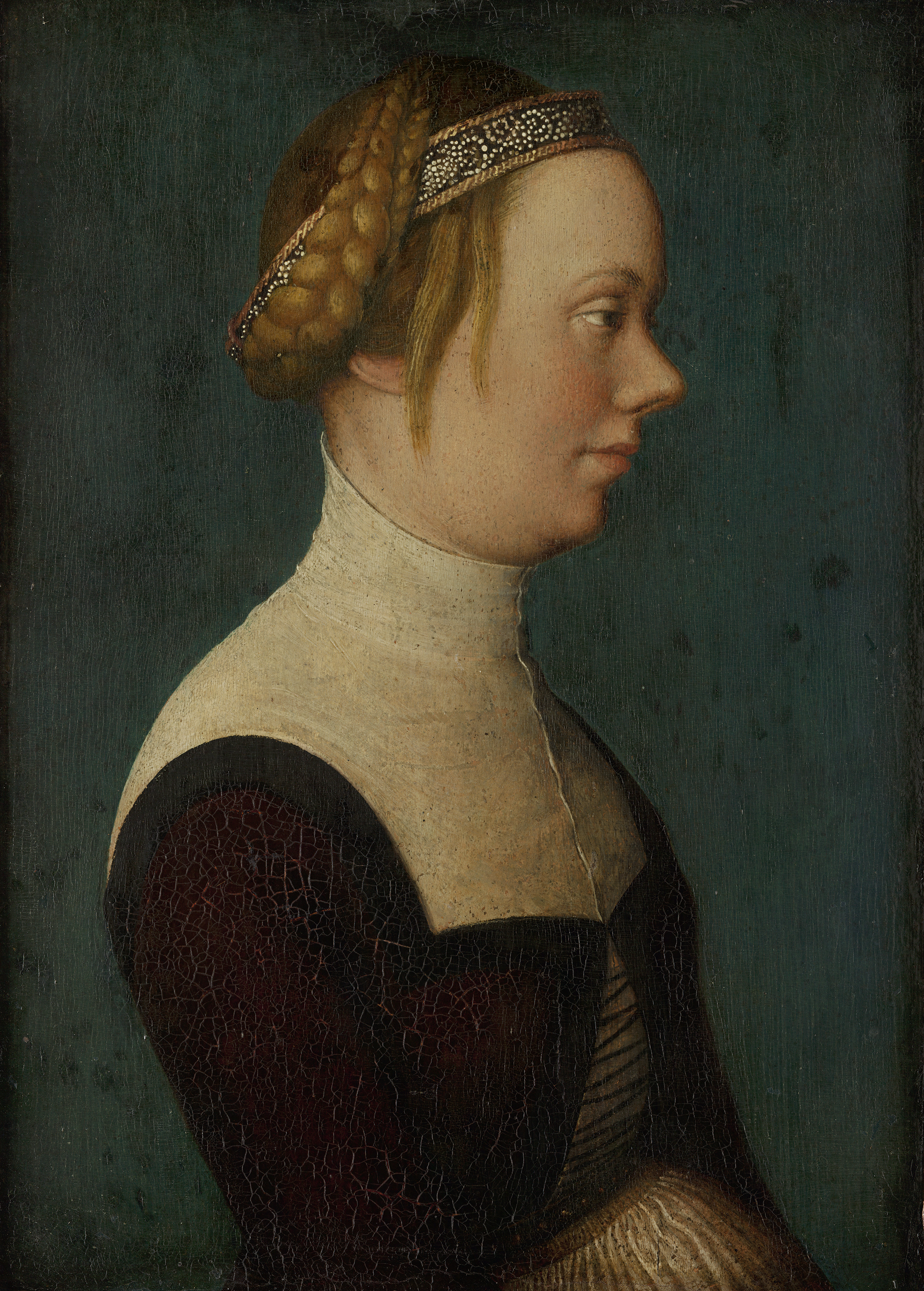This painting, reminiscent of the Dutch Masters of Antiquity, portrays a solemn and serious young woman in profile, viewed from the right side. With light tan skin, she gazes towards the right, her lips pursed and her expression stern. Her hair is a blondish-yellow, styled into a braid that is wrapped around to the top of her head, with a few tendrils cascading down the right side. She wears a jeweled headband adorned with small pearls and a braided gold rope edge, positioned just above her forehead. Her outfit consists of a white turtleneck underneath a tightly fastened, off-shoulder burgundy corset, extending up to her neck. A rounded protrusion in the lower part of the image suggests that the woman might be pregnant. She stands against a blue-gray background, with some minor cracks visible in the paint, accentuating the aged and classical style of this artwork.